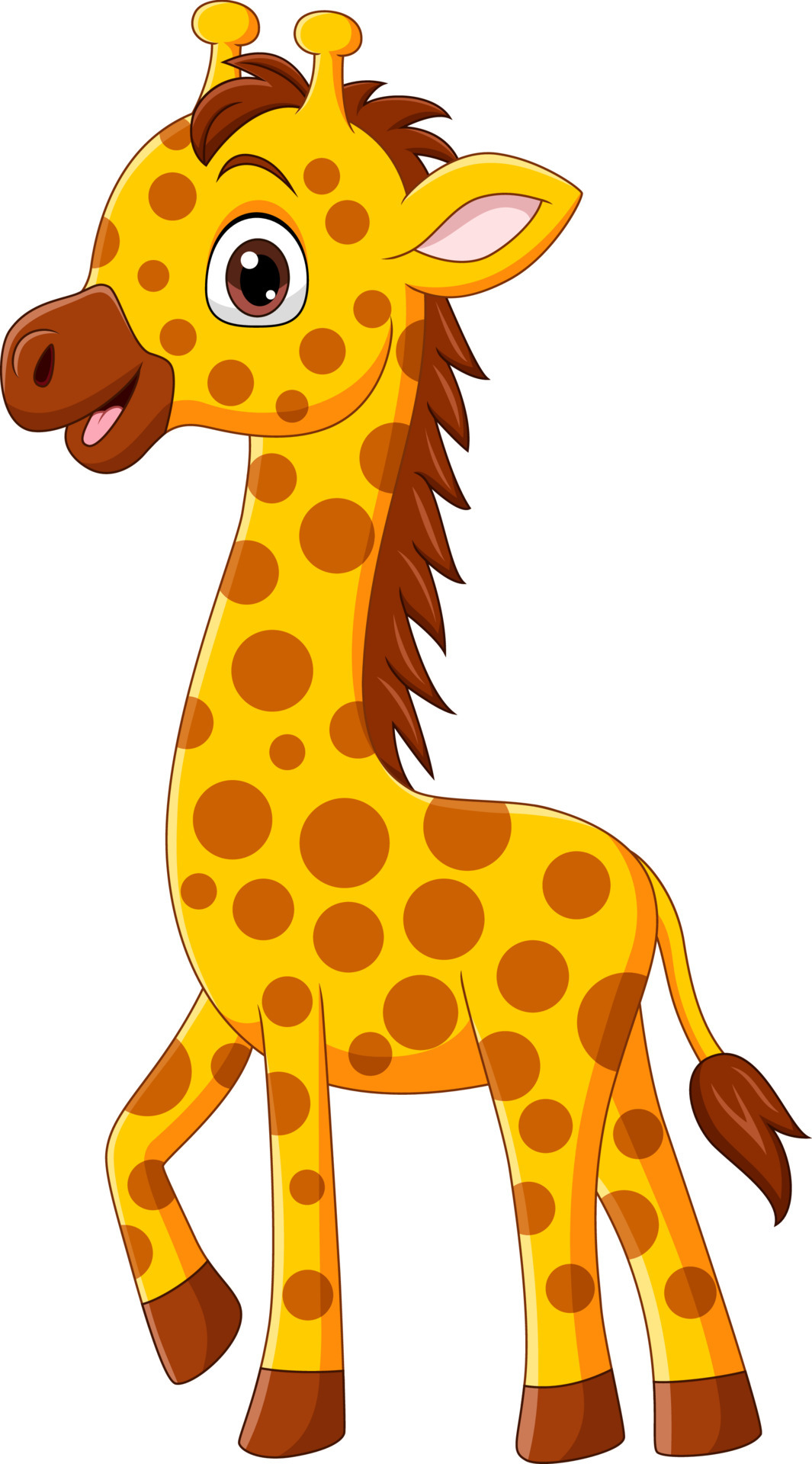This cartoon-style digital image depicts a baby giraffe marching from right to left on a white background. The giraffe, rendered in an infantile decor style, showcases bright mustard-yellow coloring with numerous uniform, circular light brown spots covering its body. It has a cheerful expression, with a raised left eye facing the viewer, a small brown nose, and a smiling mouth with a visible white tongue. The giraffe's dark brown mane extends from between its ears, down the back of its neck, and reaches its back. Additionally, it features dark brown hooves, as well as a yellow tail ending in dark brown hair. The giraffe's front right leg is lifted mid-step, giving the impression of a playful march. Its overall appearance is vibrant and endearing, perfectly suited for children's depiction.